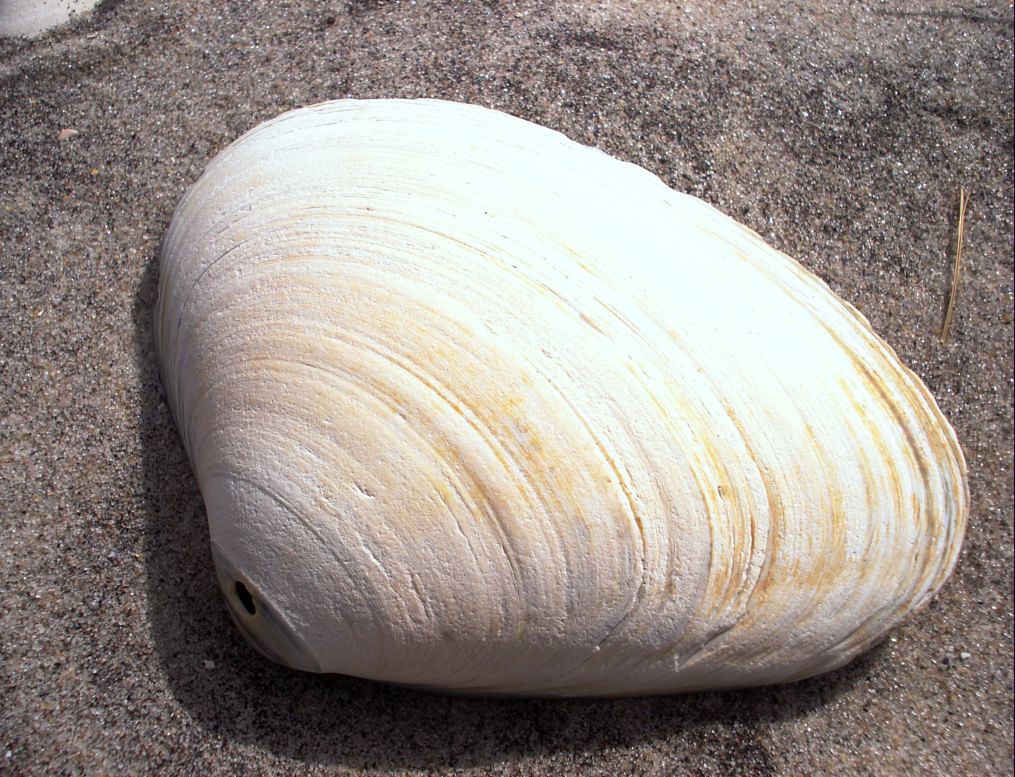This square image is a very close-up view of a large, arch-shaped seashell set against a predominantly gray, sandy background that gives an impression of being outdoors, possibly at a beach. The shell itself is primarily white with distinctive brown streaks along the upper part, the right side, and the bottom right. The surface around the shell appears textured, resembling blackish-gray sand or rocky particles. The seashell, positioned almost exactly in the center, has curved lines running horizontally and vertically, adding to its rounded triangular shape. There is a notable small hole at the top of the shell, which is partially covered with sand and dirt. The entirety of the background is gray-toned, creating a stark contrast that makes the seashell stand out prominently. The photo, devoid of any text, captures a simple yet detailed close-up of this natural object.